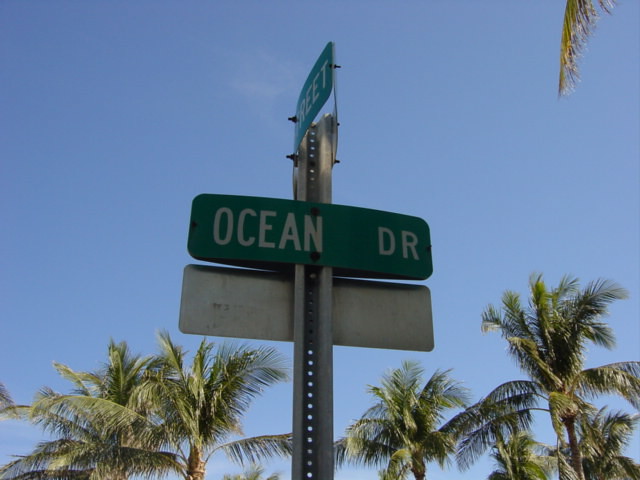This photograph captures a close-up view of a street sign on a clear, sunny day, with a vibrant blue sky dominating the background. A row of approximately six or seven palm trees with their tops stretching from the left to the right along the lower part of the image, adds a tropical vibe to the scene. A single palm frond intrudes from the top edge, contributing to the natural framing. The main subject is a metal post extending upward from the bottom of the frame, supporting three signs. The foremost sign is a green, horizontally rectangular sign with white lettering that reads "Ocean Drive." Just above this, there is another green sign only partially visible, revealing the last four letters "REET," suggesting it denotes a cross street. The bottom sign, positioned perpendicular to the Ocean Drive sign, is silver-colored and only its back is visible. The image is taken from a slight upward angle, emphasizing the natural light and outdoor setting.